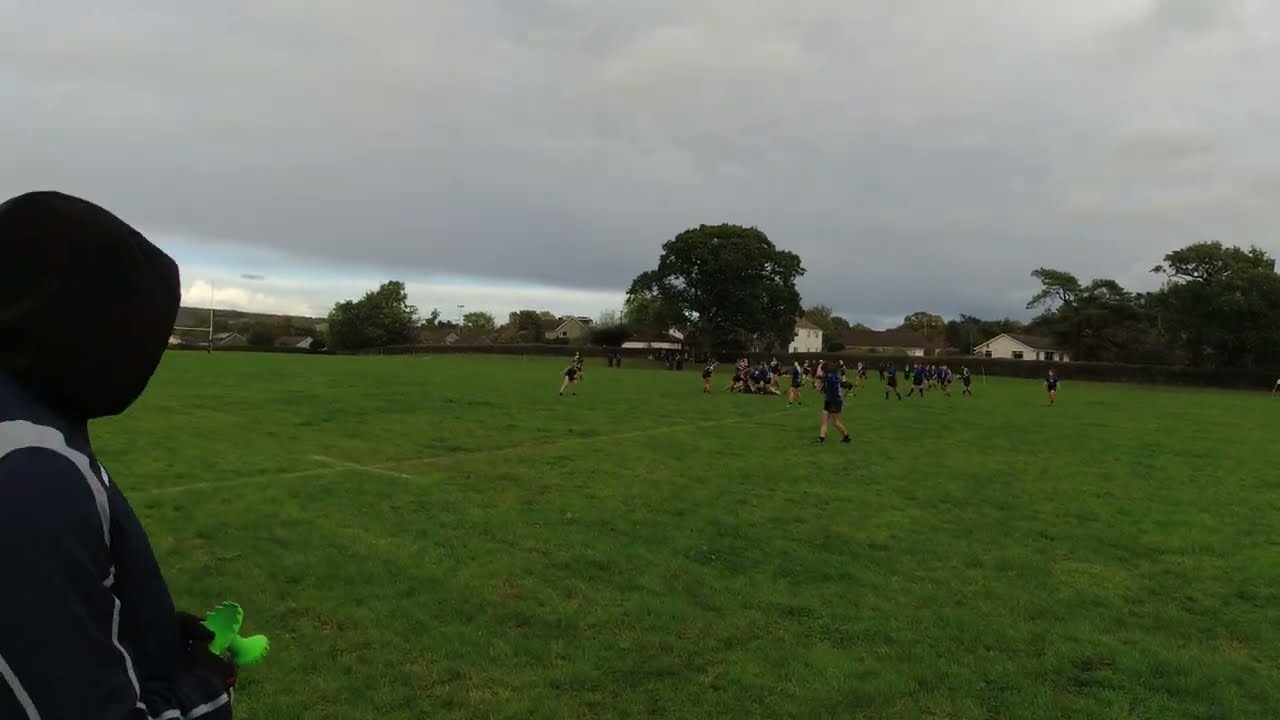In this photograph, a group of children is playing a sport, possibly soccer or lacrosse, on an overgrown grassy field. They are all dressed in blue uniforms consisting of blue shirts and shorts. The players are huddled near the center of the field, running in various directions. A faint line can be seen cutting through the grass at the center of the activity. In the bottom left corner of the image, a person—potentially a coach or referee—stands wearing a dark-colored hoodie with a gray stripe, holding a light green object that resembles a goblet. 

The background features a row of hedges, large green trees, and distant houses. One prominent house has a white wall and an arched roof, partially obscured by a large tree filled with green leaves. Another large tree extends over this house. The sky above is mostly gray and overcast, with heavy dark clouds dominating the scene, though a small patch of blue sky is visible in the distant left.